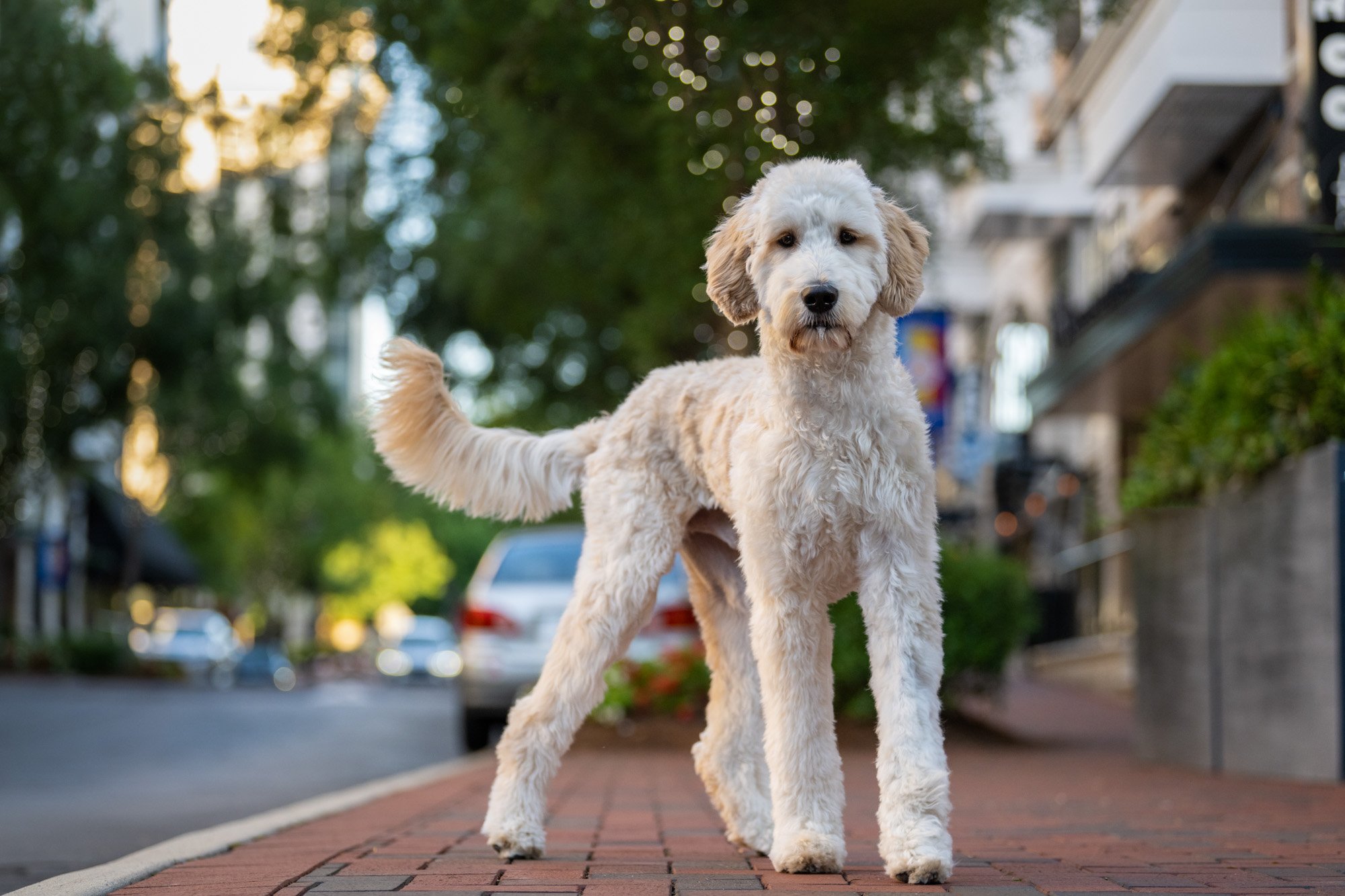In this portrait-oriented, color photograph taken during the daytime, a striking medium-to-tall white dog stands on a red brick sidewalk in a suburban neighborhood, looking directly at the viewer. The dog's scruffy, curly coat features shades of white mixed with light brown, particularly around its ears and mouth. It possesses long, tall legs and a bushy tail that curls slightly at the back. The dog has a pointed muzzle with a black nose and longish, darker beige ears. The background, slightly out of focus, reveals parked cars along the street—one being a Toyota Corolla—as well as apartment buildings on the right, shops further back, and trees overhead, adding to the suburban ambiance.